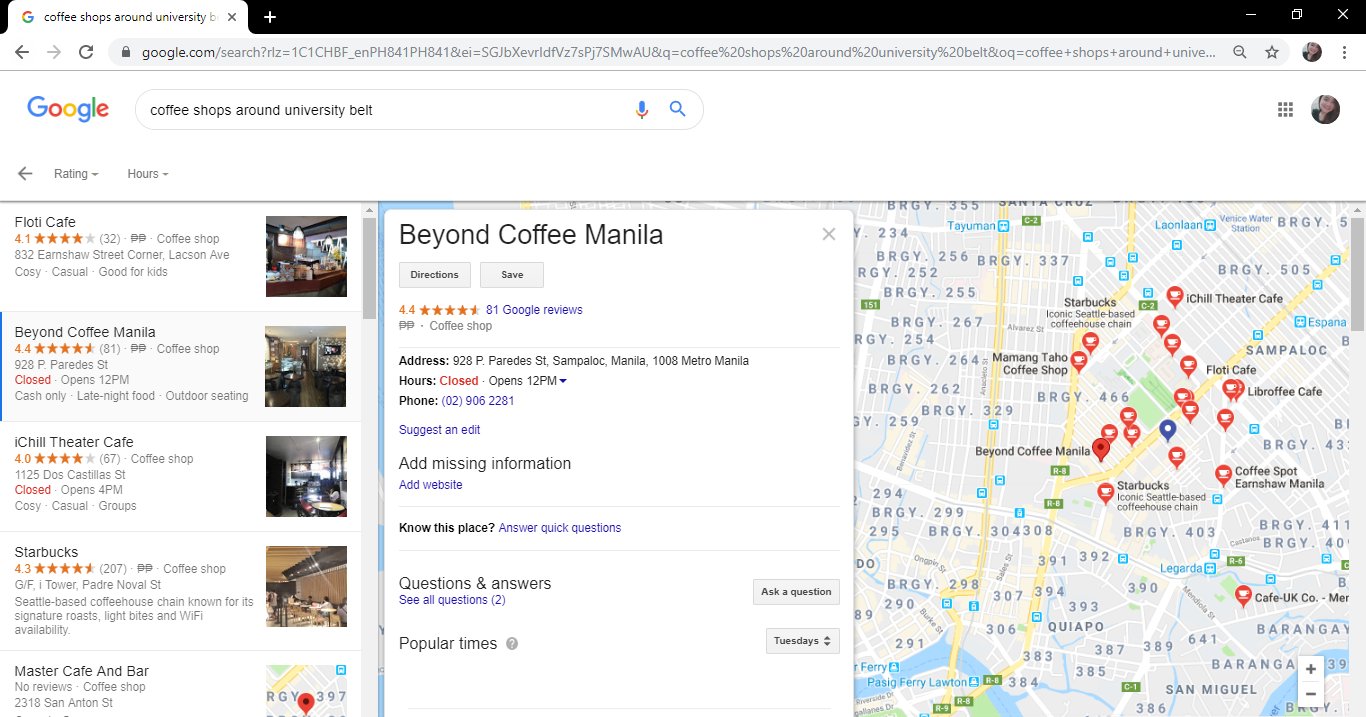This screenshot captures an organized Google search result page displayed on a computer screen. The entire interface is divided into well-structured sections for easy navigation.

At the very top, a black utility banner lies above the browser's address bar. In the upper left corner, a white tab featuring the iconic multicolored Google "G" symbol is followed by the search query in black font: "coffee shops around the university." Just below, inside a gray rectangle, is the URL link corresponding to the search.

To the far right of this section is a user's profile picture, likely that of a white female with dark hair, suggesting this is a personalized browsing session.

The main content of the screen consists of a list of search results for coffee shops around the university, organized by Google. Five coffee shop options are displayed. The first result is “Fioti Cafe” (misspelled as "Floti Cafe") with a rating of 4.1, illustrated with orange stars representing the rating; there’s also a small thumbnail image showing the cafe.

The second coffee shop listed is “Beyond Coffee Manila,” with a higher rating of 4.4 stars. Next to the name, gray text reads "coffee shop," along with the address "928P Paredes Street." A red font indicates that the cafe is "closed," while subsequent grey text states it "opens 12 p.m." A thumbnail image of the coffee shop's interior accompanies this entry. This particular result is highlighted by a vertical blue bar on its left, indicating it is the selected entry.

To the right, taking up approximately two-thirds of the screen, is an expanded view of "Beyond Coffee Manila" details. The name is prominently displayed in large letters. Directly below, options labeled "Directions" and "Save" are available. The section provides comprehensive information, including a Google Reviews link, address, hours, phone number, a "Questions and Answers" link, and a section marked "Popular times" with an adjacent question mark. Additionally, a map displaying at least a dozen coffee shop icons across the city and surrounding area is included. Among these, "Beyond Coffee Manila" is marked with a larger red icon, signifying its selection. Other visible coffee shop markers include well-known names like Starbucks, iChill Theater Cafe, and Manning Tahoe Coffee Shop.

Finally, listed below "Beyond Coffee Manila" are additional coffee shops: iChill Theater Cafe, Starbucks, and Master Cafe and Bar, providing users with a variety of choices.